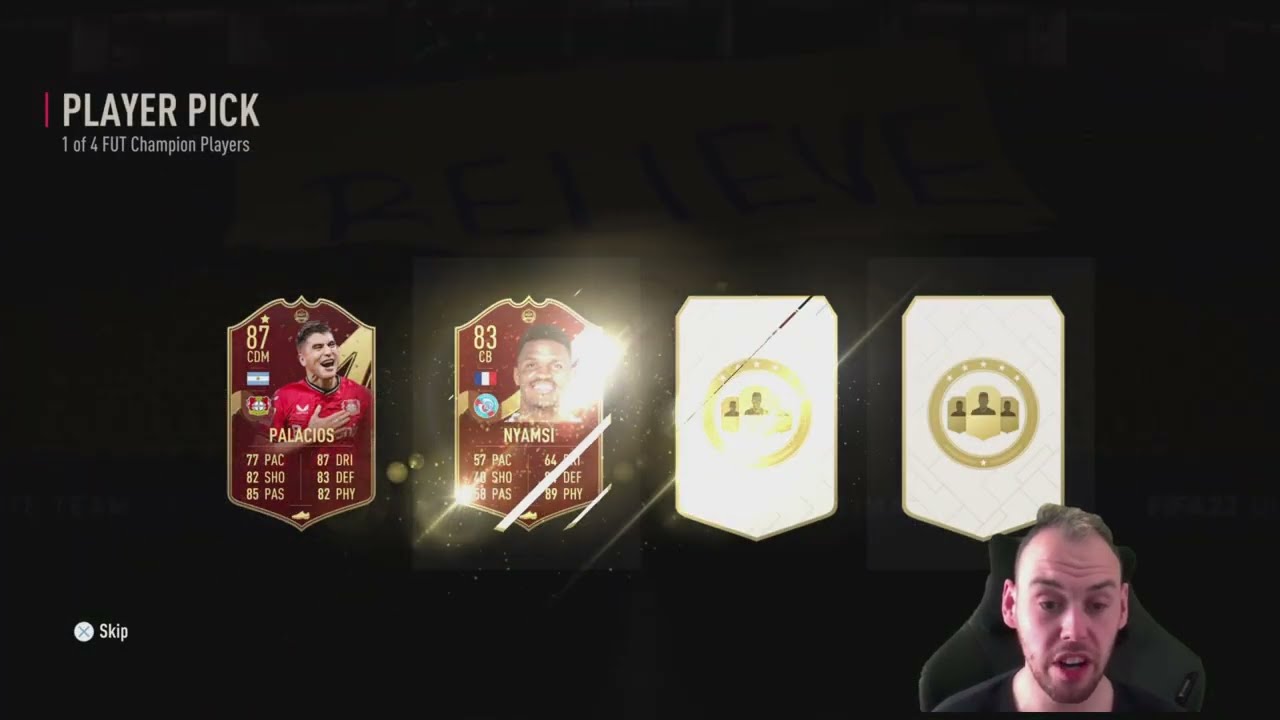The image captures a screenshot from a video where a man appears in the lower right, seated in a chair with a high backrest, and his face showing a perplexing expression as if caught mid-blink and mid-sentence. The background is predominantly black, highlighting four panels that take up the majority of the frame. These panels are labeled with player names and stats, specifically "Palacios" and "Nyamsi" with corresponding numbers indicating their ratings or attributes. Two of these panels remain unrevealed, denoted by white areas with gold rings. The top left of the image features the text "player pick one of four FUT champion players," suggesting a selection process, possibly within a fantasy soccer or betting context. The bottom left corner displays a prominent "skip" button, underscoring that this is a screen capture from an interactive video.